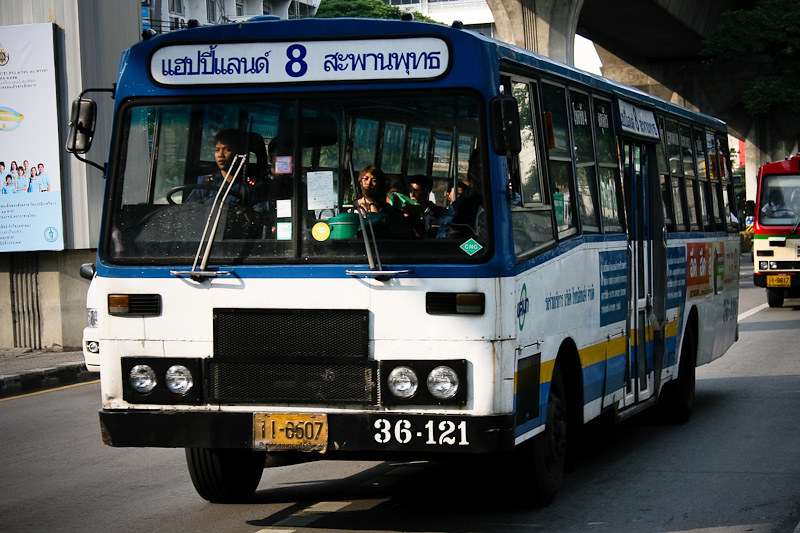This detailed close-up image depicts a somewhat old, public transit bus in a foreign country, identifiable by the driver seated on the right-hand side and indicative of a non-American setting, possibly Asian like India based on the unfamiliar writing on the bus. The bus primarily features a blue top and white bottom, with the number 8 prominently displayed on a sign atop the vehicle, while the front bumper showcases the number 36-121 in white. The bus is accompanied by another bus, following closely behind, which is distinguished by its red trim. Both buses are navigating a street under an overpass or bridge, passing by a concrete building with what seems to be individual apartments. The bus, marked with a distinctive gold-colored license plate, has large windows through which the bus driver and several passengers are visible. The antiquated design includes double doors on the side, noticeable compartments where doors close, and windshield wipers sticking upright.